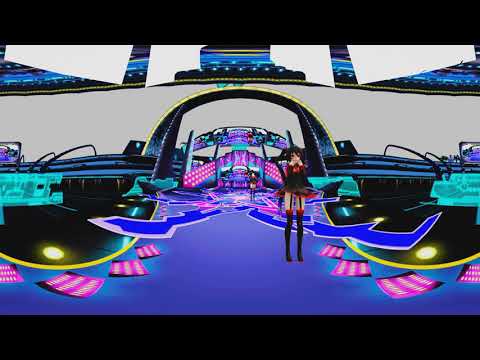This image strikingly captures a digitally generated scene, possibly from a video game, rendered in a distinctive metaverse style with fisheye distortion. It features a prominently depicted anime-style avatar of a young Japanese girl with dark hair, wearing a black and red dress or very short skirt, paired with tall boots or garters. She stands on the right side of the scene with her arms held up near her face.

The background is a vibrant neon landscape, dominated by a large black archway with yellow trim, underneath which spans another arch-like structure. Enhanced by digital elements, the environment includes scattered pink squares of light and geometric black designs on both the left and right sides, accentuated by areas of yellow light.

Towards the top of the image, a gray band stretches across from left to right, overlayed with stylized blue and black designs, as well as grayish-white rectangular shapes extending off the frame. The mid-background showcases a blue performance stage with blue lines radiating out from a pink star on the floor, suggesting a dynamic, concert-like atmosphere. Further enhancing the scene are blue spikes and purple lights creating a runway effect, adding to the digital screens and signs interspersed throughout the stadium-like environment, all contributing to the overall futuristic aesthetic.